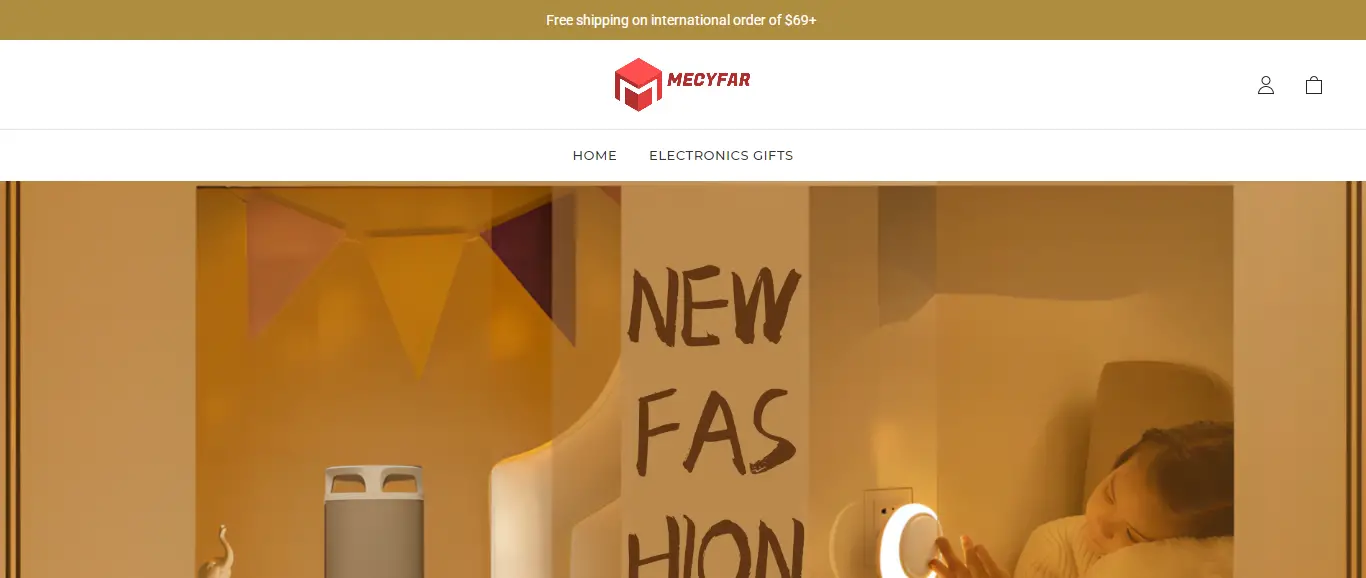The image showcases the top half of a screenshot from an online storefront. At the very top, a brown bar features white text declaring, "Free shipping on international orders of $69 plus." Below this, a white bar prominently displays the store name "MECYFAR" in bold, capitalized red letters. Positioned to the left of the store name is the store logo: a red cube with a white "M" on its side. To the right of the store logo are two icons—a silhouette of a person, presumably for accessing a user profile, and a shopping cart.

A thin gray line separates these elements from the navigation text that reads "Home" and "Electronic Gifts." Below this section is the top half of a photograph depicting a young girl thoughtfully touching a nightlight that is plugged into a wall. The wall itself has the words "New Fashion" appearing as though they were hand-painted, positioned to the right of the nightlight. The entire image is bathed in a light brown tinge, giving it a warm, vintage feel.